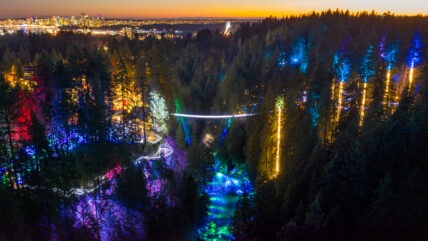The image depicts a magical and colorful mountain landscape at either dawn or dusk. The scene features a forest of pine trees illuminated with an array of vibrant lights, including hues of gold, blue, pink, red, and various shades of purple and green. On the right side of the image, five trees are adorned with yellow lights tracing their trunks, topped with blue lights at their peaks. The left side showcases additional colors, creating a visually captivating display. Nestled between the illuminated trees is a valley bathed in blue light. In the background, a brightly lit city can be seen, contrasting with the serene ambiance of the forest. The sky glows with shades of gold, orange, and red, hinting at the sun either just rising or setting, adding to the enchanting atmosphere of the scene.